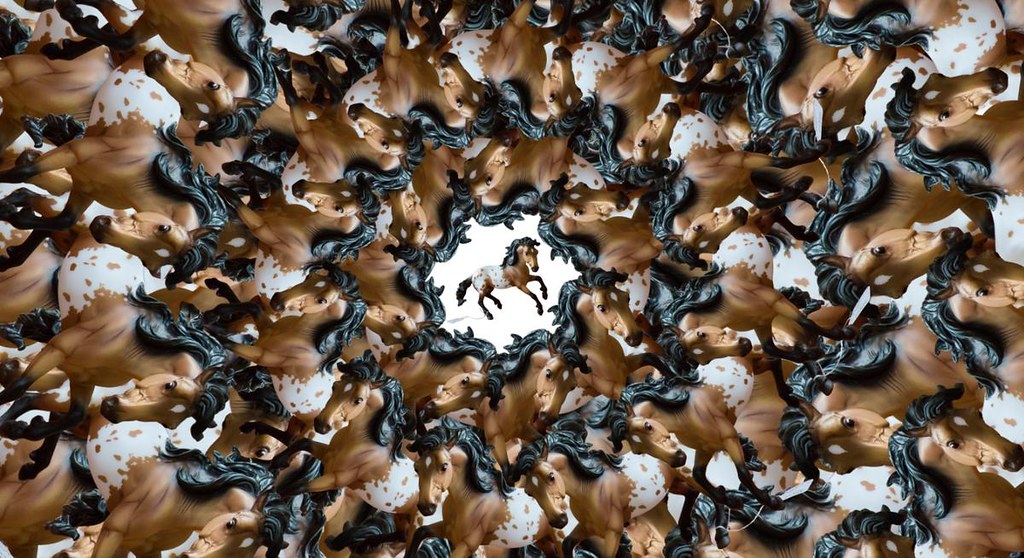The image depicts a striking arrangement of horses with a white background. At the center of the image is a unique brown horse, characterized by its black mane, black nose, and white back speckled with brown. This central horse is galloping, as indicated by its black hooves and tail. Surrounding this central horse are several more horses with identical coloring and features, forming concentric circles around it. Their black manes collectively create multiple radiating black circles, making the composition more dynamic. Each horse's front is brown with a black mane, face, and hooves, while their hindquarters are white with brown freckles. The organized layers of these horses, spiraling inward, create a captivating visual of unity and motion.